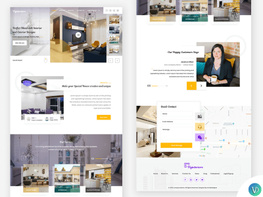The image is divided into two sections, each containing multiple pictures. The content is somewhat blurry, but discernible.

### Right Section:
1. **Top Section**: Features three images showcasing room interiors. These images display couches, tables, and cabinets.
2. **Middle Section**: Shows a woman in a black suit holding a white cup of coffee. She is seated on a yellow couch, with a partially readable black text on a white background to her left. 
3. **Bottom Section**: Contains a sign-up form that asks for an email, first name, and second name. Below this form, there is a map.

In the bottom right corner, there is a circular icon with a green and bluish fused background, containing a white "V".

### Left Section:
1. **Top Section**: Displays an image of a room interior with white and black walls and yellow chairs.
2. **Bottom Section**: Features three pictures of house exteriors, all of which are brown.

The left side and right side images are neatly organized and present a blend of interior and exterior views.